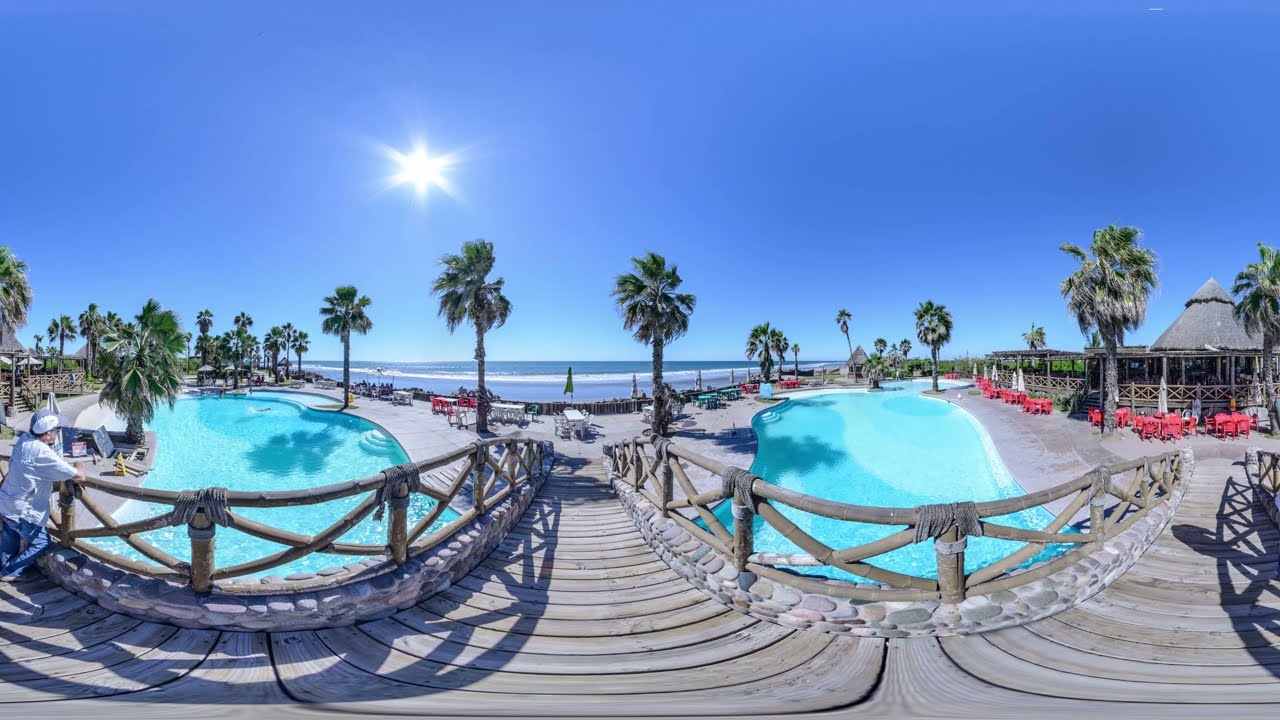This panoramic image captures a vibrant beachside resort against the backdrop of a stunning deep blue ocean and a clear, blue sky. The horizon is centrally placed, with the sun slightly to the left, creating a visually striking six-pointed star shape in the sky. The foreground of the image features two kidney-shaped swimming pools filled with turquoise water, flanking a rustic, gray wooden walkway with railings. To the right, a charming beach bar with a triangular thatched roof is surrounded by a mix of red, white, and blue plastic chairs and tables, some of which have outdoor umbrellas. On the left, a man wearing jeans, a casual shirt, and a baseball cap leans against the railing, gazing over one of the pools. The resort is enveloped by trees reminiscent of palm trees, suggesting a likely Mediterranean location.